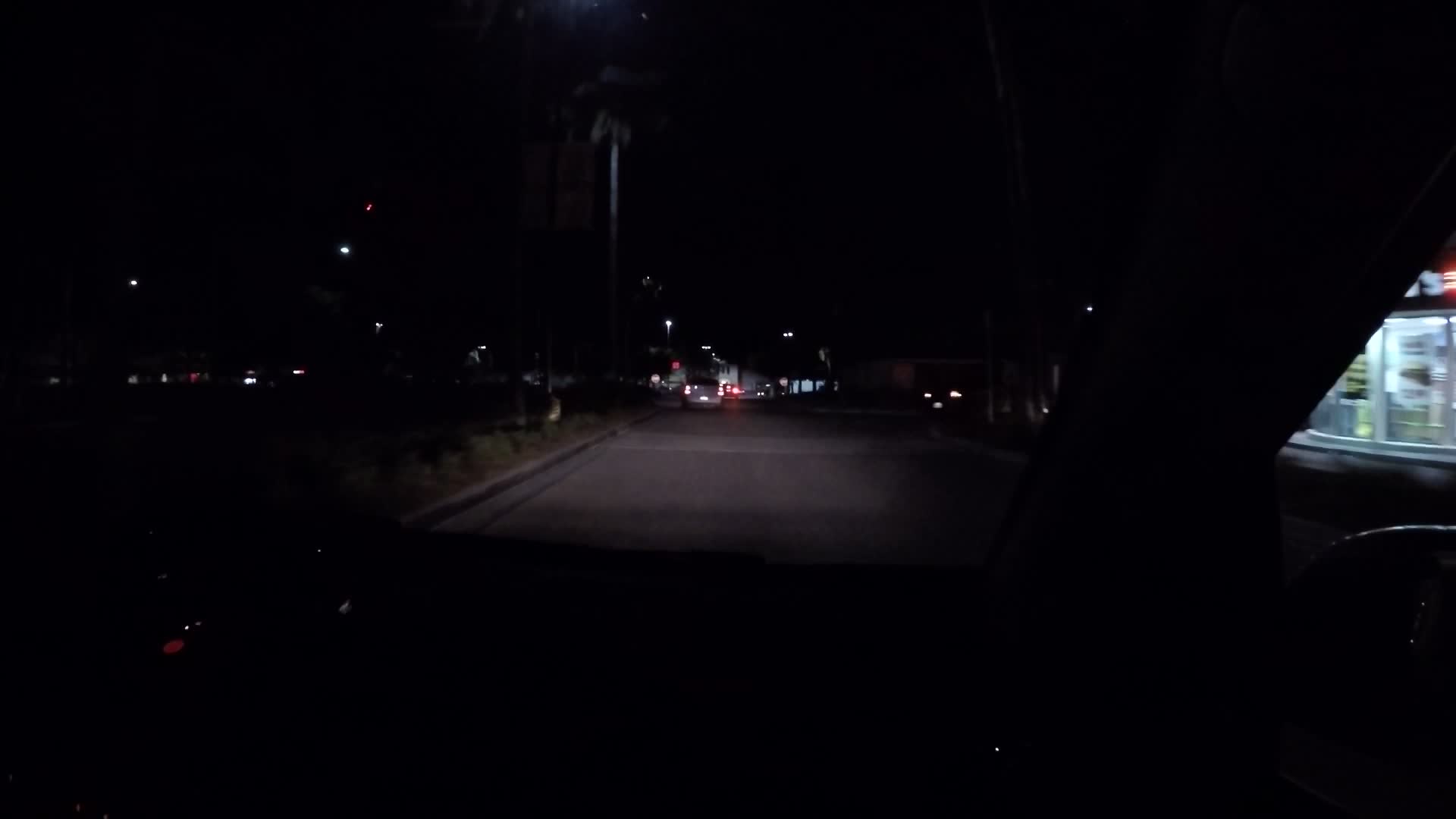This nighttime photo, taken from inside a vehicle, captures a poorly lit scene with minimal illumination. The bottom portion of the image is mostly engulfed in darkness, except for a faint reflection on the right side that hints at the presence of a steering wheel. Beyond this, the road ahead is shrouded in darkness, interrupted only by a single glowing street light that casts a small pool of light onto the asphalt, creating a stark contrast with the pitch-black surroundings. In the distance, brake lights and subtle vehicle lights from cars further ahead are visible, contributing to the sparse illumination. To the right, beyond the car's window, a brightly lit convenience store with large glass windows stands out, adding a distinct point of interest. Scattered faint lights dot the horizon on the left, adding depth to the otherwise shadowy landscape. The overall composition emphasizes the isolation and obscurity of the night, with sporadic points of light providing the only reference points in the encompassing darkness.